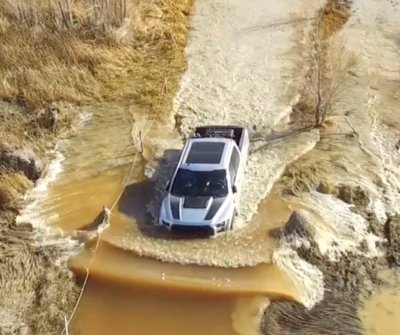This photograph captures a detailed scene of a relatively low-resolution image (about 200 by 300 pixels) showing a white, new, and clean truck driving through deep floodwaters that reach almost to the top of its hood and around its headlights. The truck is prominently positioned in the center of the image and appears to be a mix between a pickup truck and an SUV. It features black geometric shapes on the front, a black sunroof, dark windshield, and a black bed. The vehicle is navigating through muddy, brownish-yellow water, which is opaque and turbulent, indicating movement and speed. A significant wake and splashes are visible around the truck, suggesting it is displacing a considerable amount of water while driving. The fore and background show a wake of white-tipped waves trailing behind the truck. 

The surrounding environment seems desolate, characterized by pushed-back grass along the sides from the floodwaters, and the field extending beyond the water is full of dirt and dead, brown grass. The scene likely depicts a rural area with no visible people or text in the photograph. This image was captured during the daytime, offering a clear view of the truck's struggle through what appears to be a canal or ditch filled with floodwater.